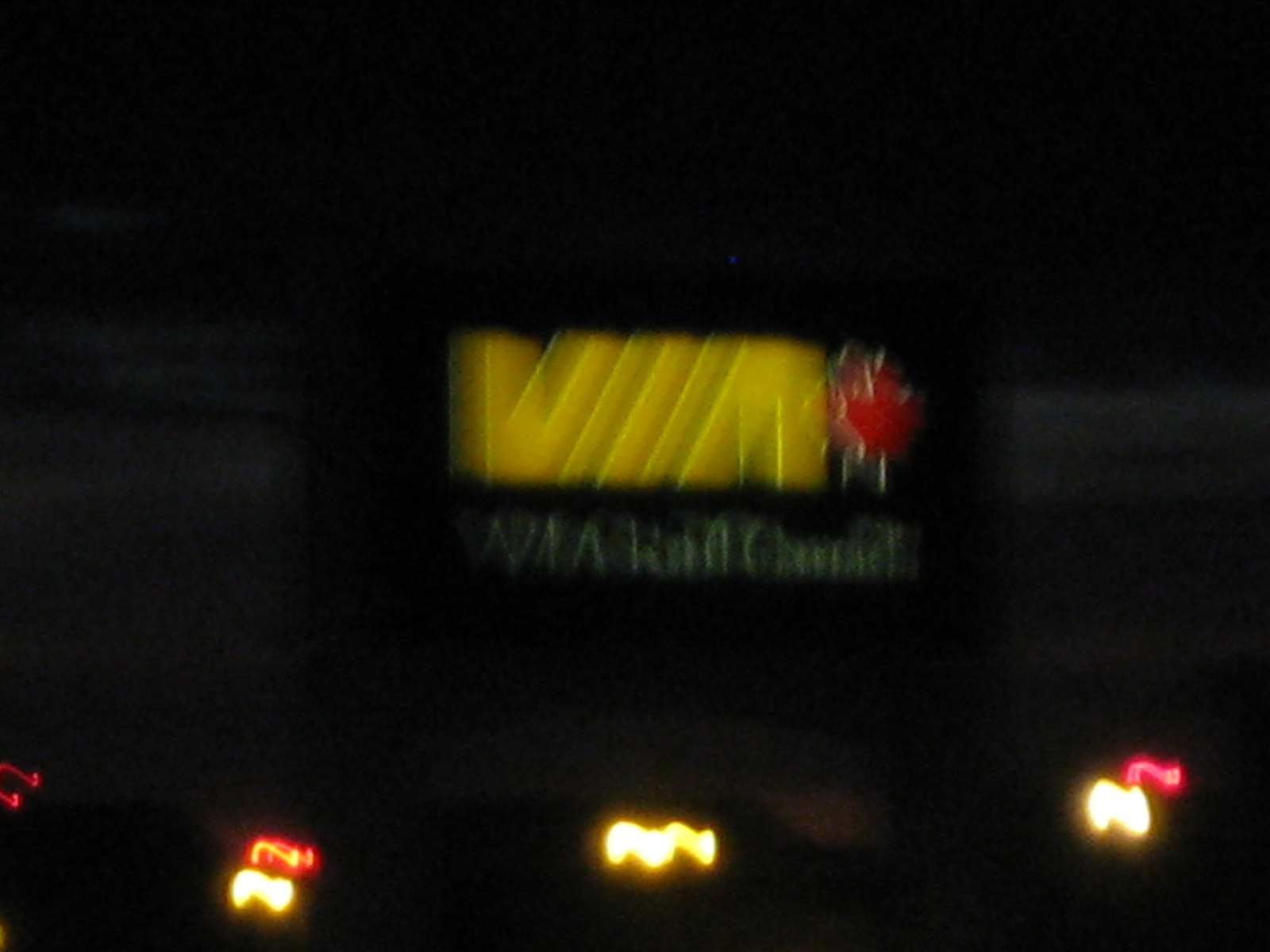The image depicts a nighttime scene taken while in motion, resulting in a very blurry photograph of a sign. The background is black, and at the center of the sign, there are yellow neon characters that resemble a "W" followed by three sideway eyes or backslashes, and then what might be an "M," though it's highly unclear. To the right of these yellow characters lies a red, spiked ball-like shape, described variably as a berry or just a small red dot. Below the yellow text, there's green text which is extremely difficult to decipher but appears to spell something like "WIA" or "VIA Channel." At the bottom of the image, three bright lights are visible, with some observers noting these lights have a red Z-shaped form on top or resemble apples with red stems. All elements of the image are significantly blurred.